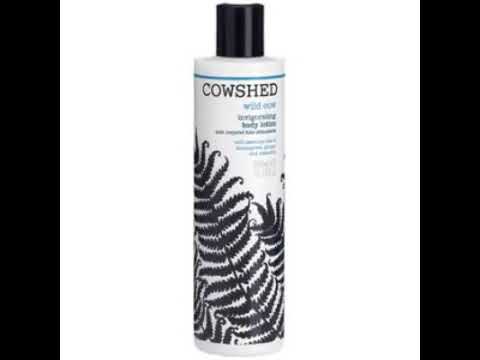The image depicts a tall, cylindrical bottle standing upright at the center of a white square background. The bottle, likely a product like shampoo, is primarily white with a black leafy design adorning its surface. This intricate design, resembling delicate fern leaves, starts at the bottom right side and extends upward, with jagged curly leaves branching out from a central stem. The bottle has a sleek black cylindrical cap, accented with a thin blue band beneath it. The cap is flat on top, with a broader base where it screws onto the bottle. Along the top of the bottle, black uppercase text reads "COW SHED," followed by partially obscured smaller text, possibly indicating the product variant. The image is bordered on both sides by thick vertical black strips, contributing to a clean, minimalist aesthetic likely intended for commercial or stock photography purposes.